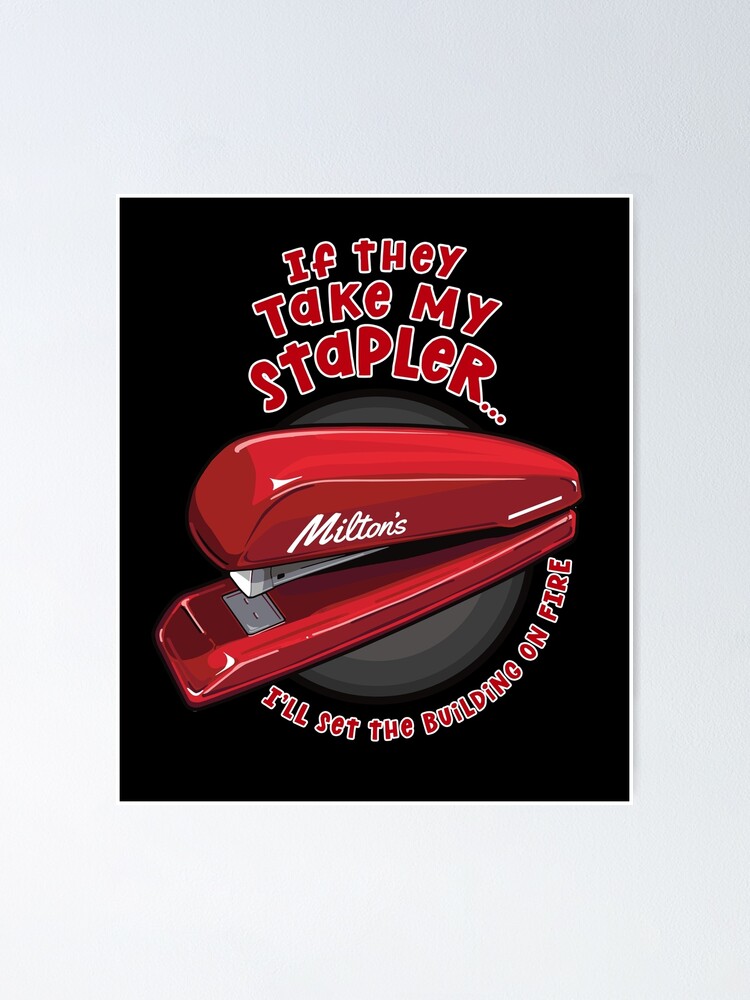The image depicts a poster-like graphic featuring a bright red stapler prominently positioned in the center. The stapler has the word "Milton's" inscribed on its side in white. Surrounding the stapler, in bold red block lettering with a thin white outline, is the text: "If they take my stapler," appearing at the top, and "I'll set the building on fire," located at the bottom. The textual elements pop against a predominantly black rectangular background, which itself is nested within a larger, solid gray background. The design and phrase reference a well-known scene from the movie "Office Space," where the character Milton expresses his attachment to his stapler. The overall style of the graphic, coupled with the humorous text, suggests it’s intended to be a playful homage to the film.